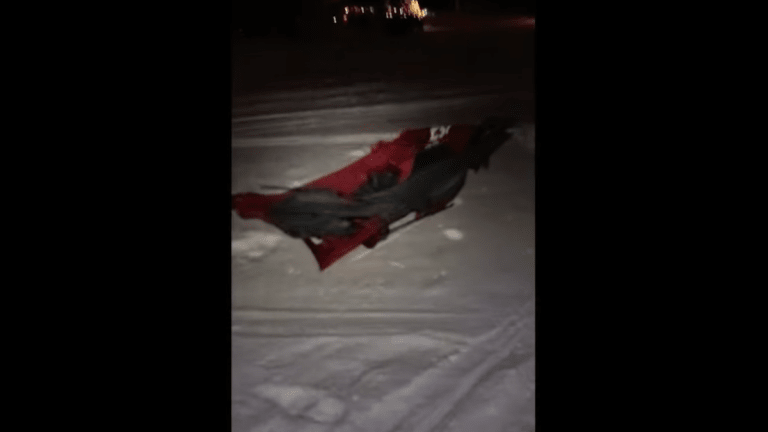The image is divided into three vertical sections, with the left and right sections completely black. The central section features a nighttime photograph of a snowy ground. Dominating the middle part of the photo is a red and black colored cloth lying on the snow, suggesting it might be a flag or a blanket. The snow-covered ground shows footprints and tire tracks around the cloth. In the distance at the top of the central section, there are small, blurred yellow and white lights that appear to be from a housing area or streetlights. The overall scene is dark and cold, with the rest of the background blending into black.